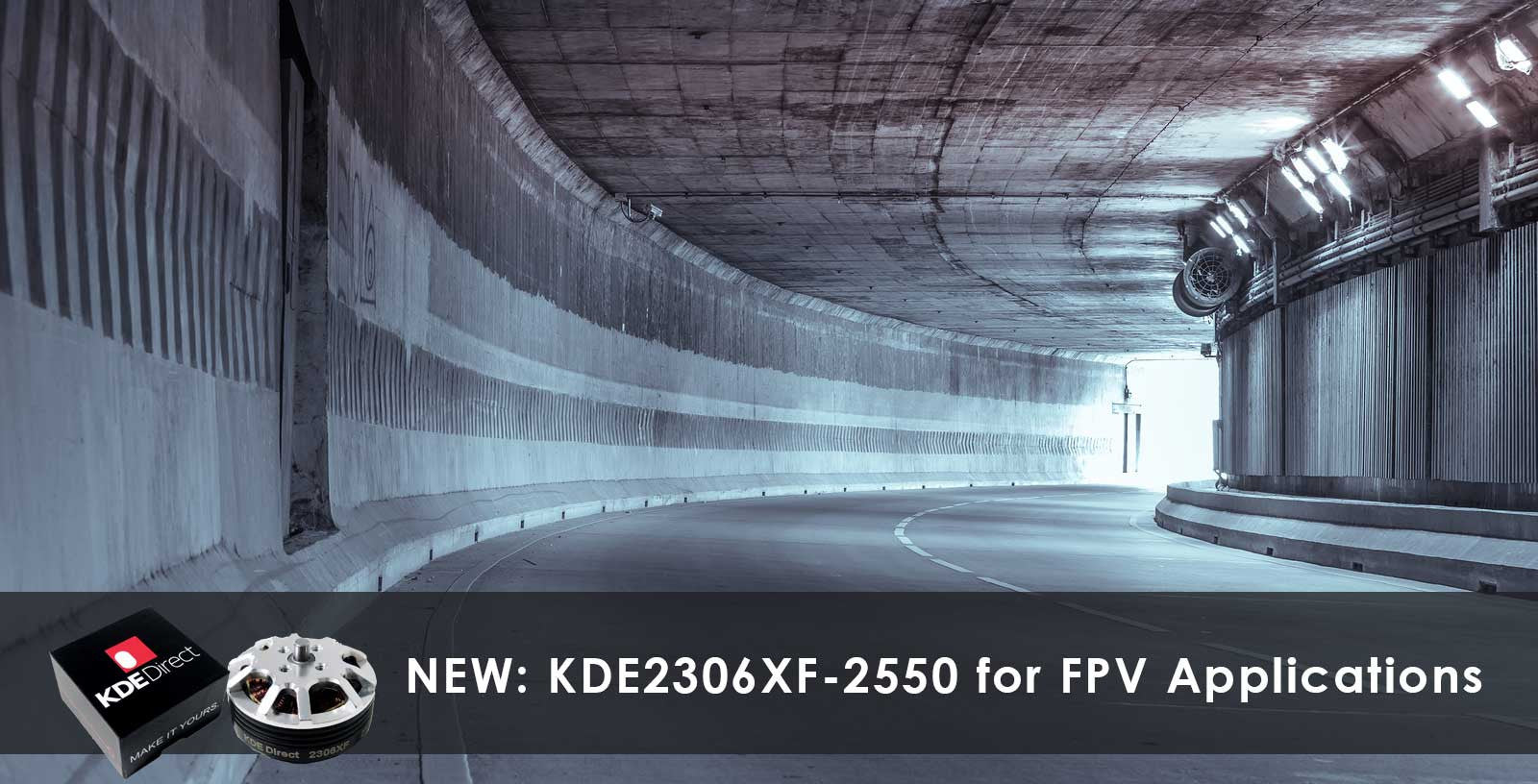The image showcases a highly detailed and realistic scene that appears to be AI-generated or derived from a video game, depicting the interior of a stark, brutalist tunnel. The tunnel features two lanes separated by a hashed yellow line, suggestive of a high-speed vehicular path with no designated pedestrian area. The left wall curves gracefully and is adorned with ridges along the middle and at the top, adding texture and a utilitarian aesthetic, characteristic of brutalist architecture. Similarly, the right wall mirrors this curvature but also includes bright white floodlights installed along the upper edge, illuminating the scene with a harsh, clear light. The ceiling above seems constructed of concrete blocks, further emphasizing the tunnel’s raw, industrial design.

In the foreground and prominently positioned is a new brushless motor identified by the text overlay as "New KDE 2306XF-2550 for FPV applications." This caption is presented within a black rectangle with white text at the bottom of the image. Accompanying the text, a white, dome-shaped motor with slots around its edges is prominently displayed. To its left, the item’s black and red container is visible, featuring the brand name KDE Direct. The image is a color photograph rendered in a style that blends photographic realism with representationalism, focusing on both the architectural elements of the tunnel and the precise detailing of the product.